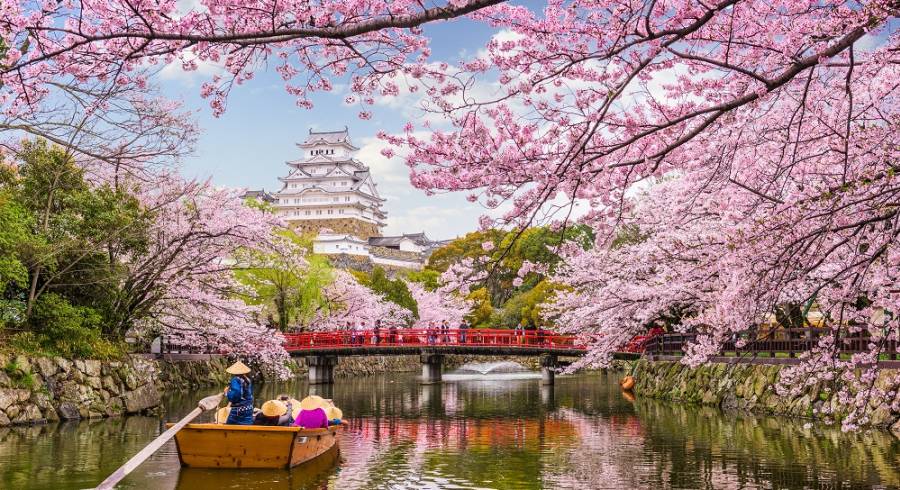The image captures a serene, picturesque canal scene that exudes the charm of traditional Asian architecture, likely set in either Japan or Vietnam. Dominating the background is an impressive multi-tiered pagoda, its beautifully white and brown structure standing majestically. In the middle ground, a graceful, orange-red bridge crosses the canal, with people leisurely walking across it, adding to the lively atmosphere.

In the foreground, the tranquil canal, reflecting the vibrant hues around it, is home to a medium-sized wooden boat. This boat, steered by a solitary oarsman clad in a blue robe, carries about six tourists, all wearing traditional pyramid-shaped hats. They glide under the bridge, enveloped in the peaceful ambiance provided by the stunning cherry blossom trees. These blossoms, in varying shades of pink, stretch out over the water, almost touching their reflections on the canal's surface.

Green trees intersperse with the blossoms, adding depth to the layers of colors that make this scene visually striking. The pristine water and the pink and white flowers framing the image evoke an inviting, tranquil vibe, perfectly suitable for a travel magazine cover. The scene's meticulous details make it a captivating portrayal of an idyllic, must-visit destination.